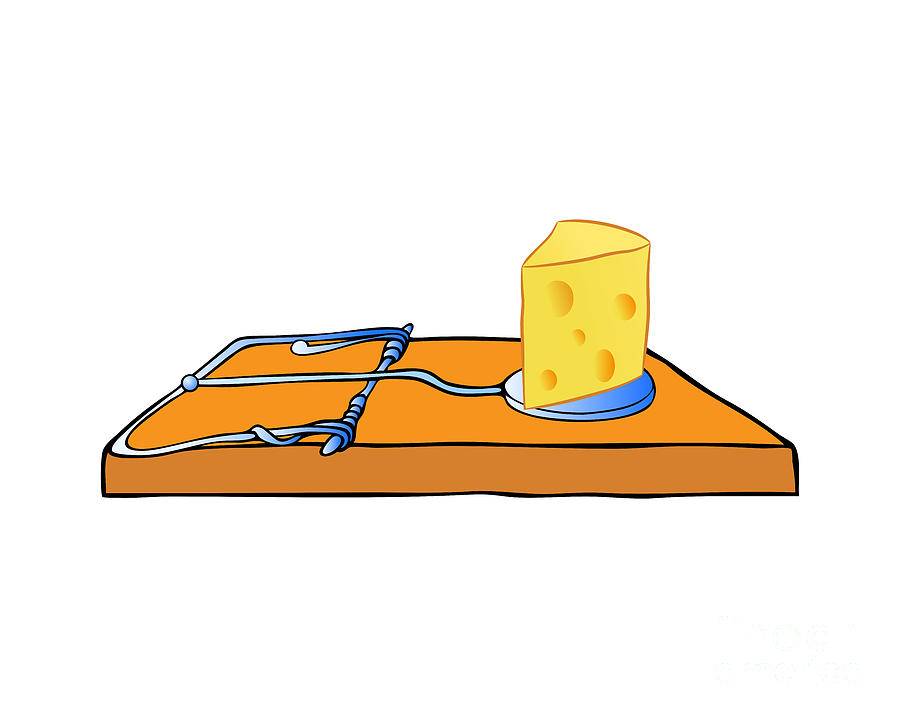The image is a detailed cartoon drawing of a classic wooden mousetrap, depicted against a plain white background. The trap is illustrated in profile, aligned horizontally at the bottom of the image. The wooden base of the trap is a brown-orange color, with a piece of Swiss cheese placed prominently on the right-hand side atop a silver-colored, round metal plate. The Swiss cheese is yellow with indicative marks to represent its characteristic holes. Extending to the left from the metal plate is a wire, part of the spring-loaded mechanism, which is fully armed and ready to spring. This wire terminates in a steel-colored ball that lies across the back left edge of the trap, securing it in place. The cartoon's lines are somewhat irregular, contributing to a sketch-like quality. The scene is devoid of any additional elements, text, or background, focusing entirely on the mousetrap and its tempting bait.